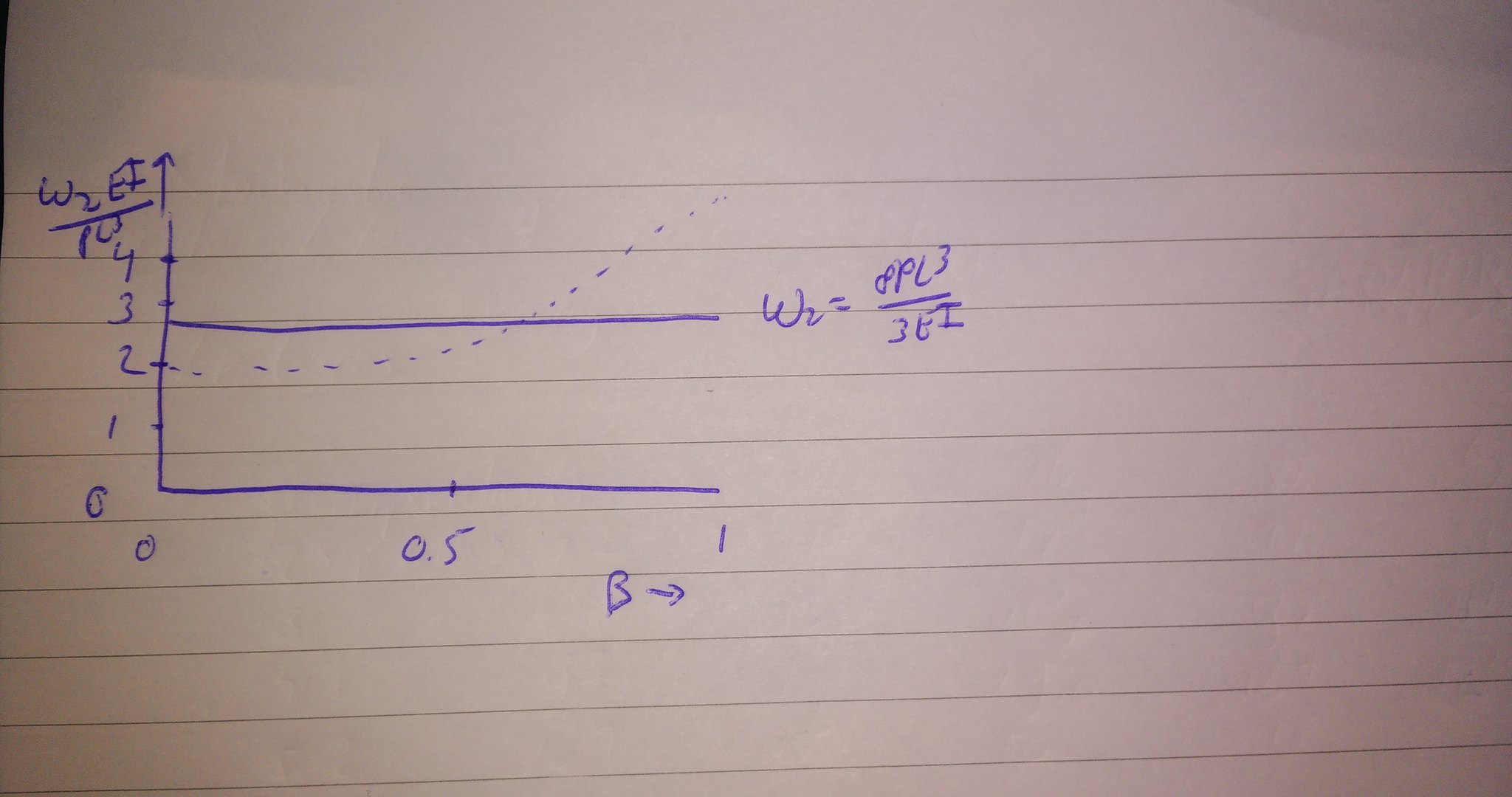This image depicts a piece of geometry homework. It features a graph with an x-axis and a y-axis. The y-axis is marked with numbers 1, 2, 3, and 4, while a line is drawn horizontally just below the number three. The graph is overlaid with a formula, "w2 = 8PL3 / 3EI," positioned to the right of the main graph area.

Additionally, there is a dotted line starting from the y-value of 2, intersecting the solid line placed under the y-value of 3. At the bottom of the graph, the x-axis is labeled with numbers starting from 0, then 0.5, and includes a 'B' with an arrow pointing to the right side of the image. This detailed setup suggests the graph is part of a complex problem, likely involving the calculations and visual representations typical in a geometry or engineering context.